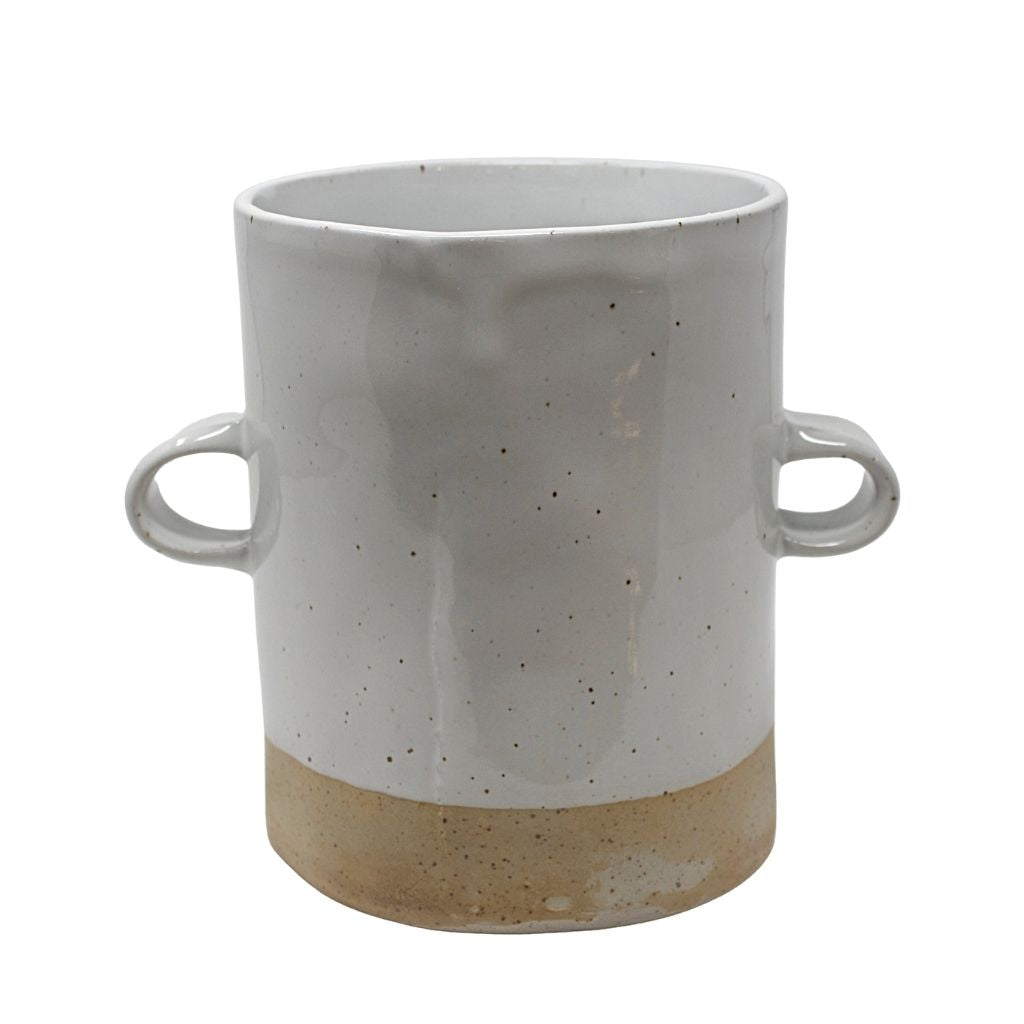This image features a handmade ceramic coffee mug, predominantly gray with a beige band encircling the bottom. The surface is adorned with black flecks, adding texture and character. Notably, the mug has two small handles on either side, a unique feature compared to traditional mugs. The top rim displays subtle drips, suggesting a handcrafted glazing process, and the interior matches the gray exterior. The object is slightly off-center in the frame, with a faint, indistinct black shadow reflected on its surface. The mug's smooth and shiny finish reinforces its artisanal origin, making it suitable for various uses, from holding beverages to organizing pencils and pens.